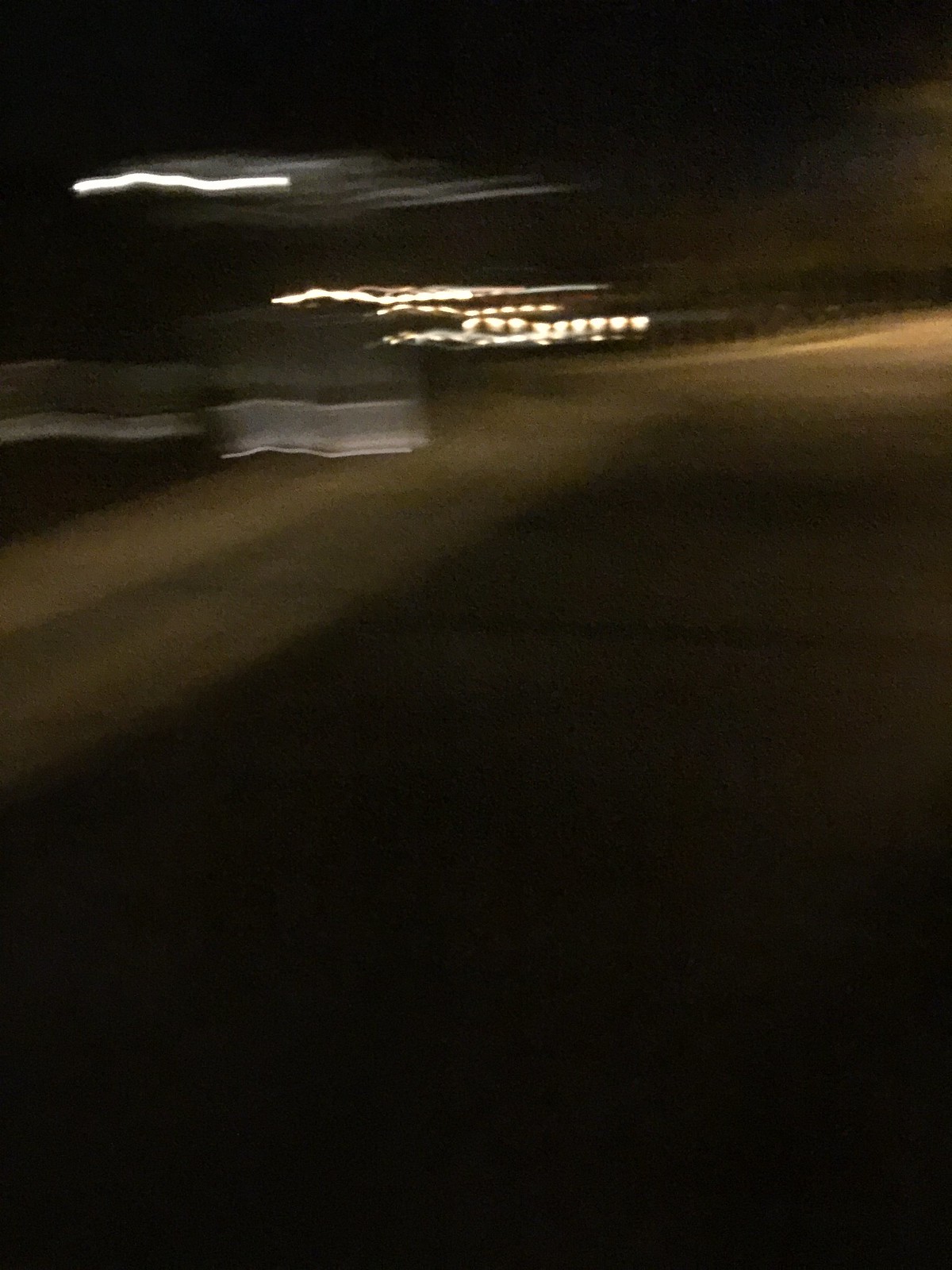This vertical rectangular photograph, taken at night, captures a dynamic motion blur of lights against a predominantly dark backdrop. The image is mostly black, with the deep black occupying the top third and bottom right corner. The bottom left corner and the top right corner are slightly lighter shades of black, adding depth to the composition. 

In the top left corner, a bright, glowing white line streaks across the frame, creating the effect of motion. Beneath this, there are dotted lines and squiggly paths of light in a light yellow or cream color, contributing to the overall ethereal atmosphere. These lines appear to be in motion, likely due to the camera being moved during the shot, resulting in ghostly trails and shadows. 

A subtle hazy line of light, running horizontally about a third of the way down, further divides the composition into distinct sections. Below this hazy line and in the center of the photograph, faint brown tones suggest the presence of a road or another ground surface, although it remains blurred and indistinct. This brown area extends from the middle left side towards the right, fading into the darkness. 

Overall, the image evokes a sense of nighttime movement and the transient nature of light in a dimly lit street, creating an almost abstract rendering of motion and luminosity.